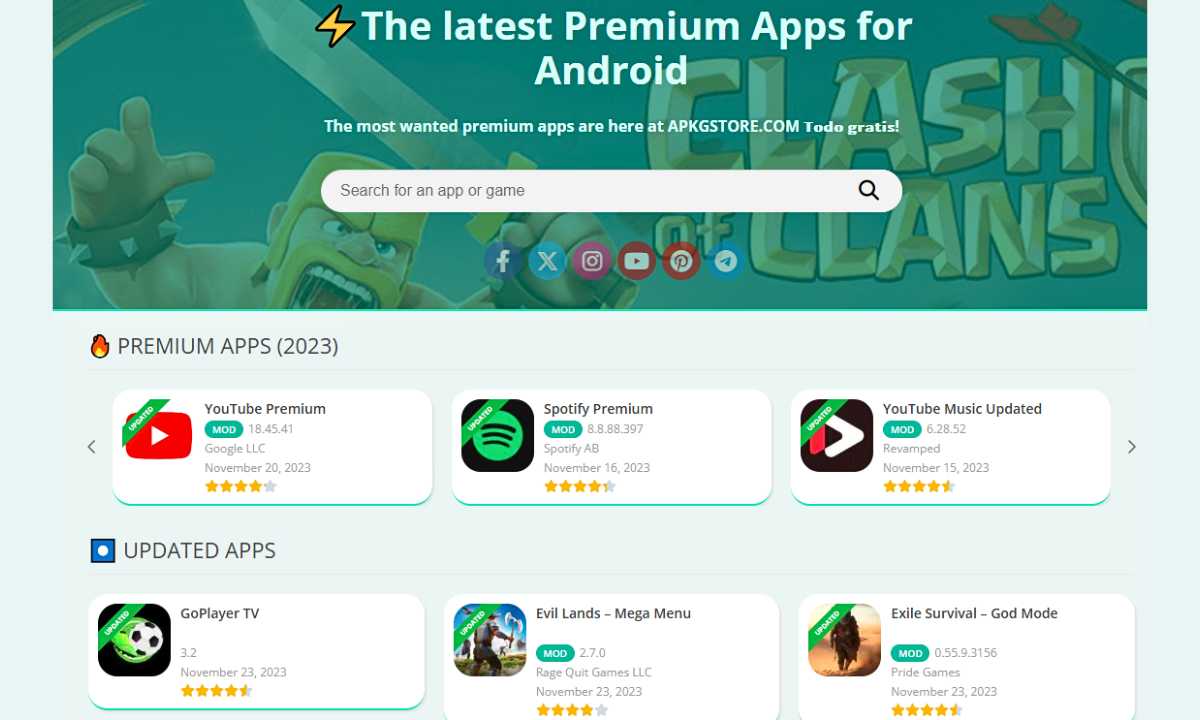*The image depicts a bustling digital marketplace interface, specifically a screenshot from the premium app APKG Store. The main section showcases a prominently highlighted app, "Clash of Clans," with striking yellow text on a dark background. Beside it, a character is depicted wielding a sword and wearing a spiked bracelet, anchoring attention to its offering of "Fire Premium" for $20.03. Below, the interface features options for Facebook, Twitter, Instagram, YouTube, and Pinterest icons, providing easy access to these social platforms.*

*Adjacent listings include "YouTube Premium" indicated with blue text and a four-star rating, and "Spotify Premium," also bearing a distinct four-star rating symbol. We're presented with "YouTube Music Updated," rated at 4.5 stars, as well as "GoPlayerTV," similarly rated at 4.5 stars under the "Updated Apps" section. Further down, there's a preview of other applications such as "Equalance," "Mega Menu," and "WhatsApp." A specific mention of "Exile Survival" is noted, along with its version number, November 23.3, boasting a 4.5-star rating. In the bottom corner, an ambiguous figure of a person suggests user-centric interactions or maybe a promotional character within the app's environment.*